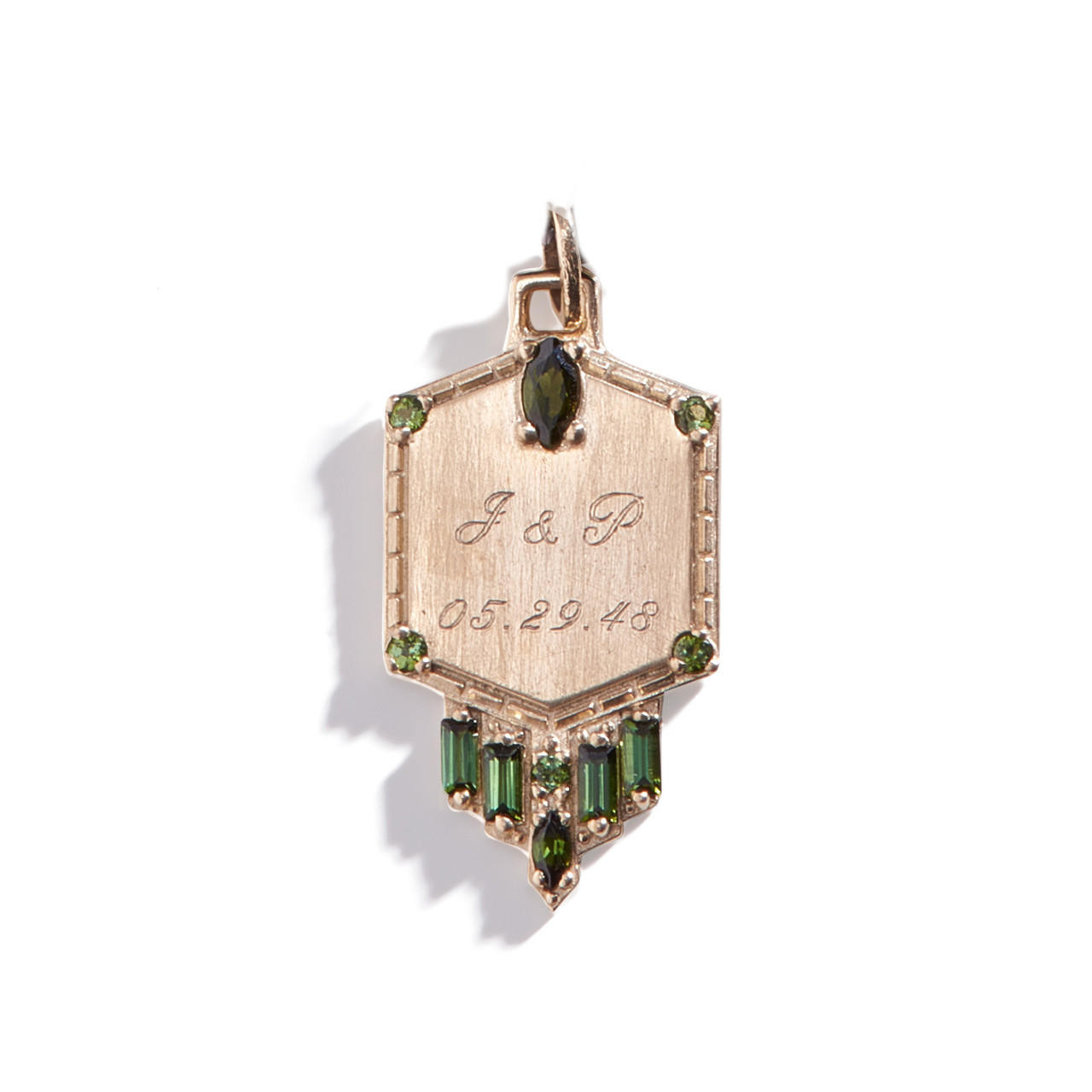This image depicts a hexagonal gold pendant, placed against a solid white background. The pendant appears to be made of wood with a subtle vertical grain, displayed in a light to medium shade. Its hexagonal shape features elongated left and right sides compared to the shorter top and bottom sides. In the center, the letters "J&P" are intricately inscribed in a script font, followed by the date "05.29.48" beneath them. At each of the four corners sits a small green gemstone, likely emeralds. Dangling from the bottom of the pendant are five additional green stones: four rectangular and one oval. A larger marquise-cut green gemstone is positioned at the top of the pendant, just below the attachment loop, which currently lacks a chain. The pendant casts a shadow to the left, enhancing its three-dimensional appearance on the clean white surface.